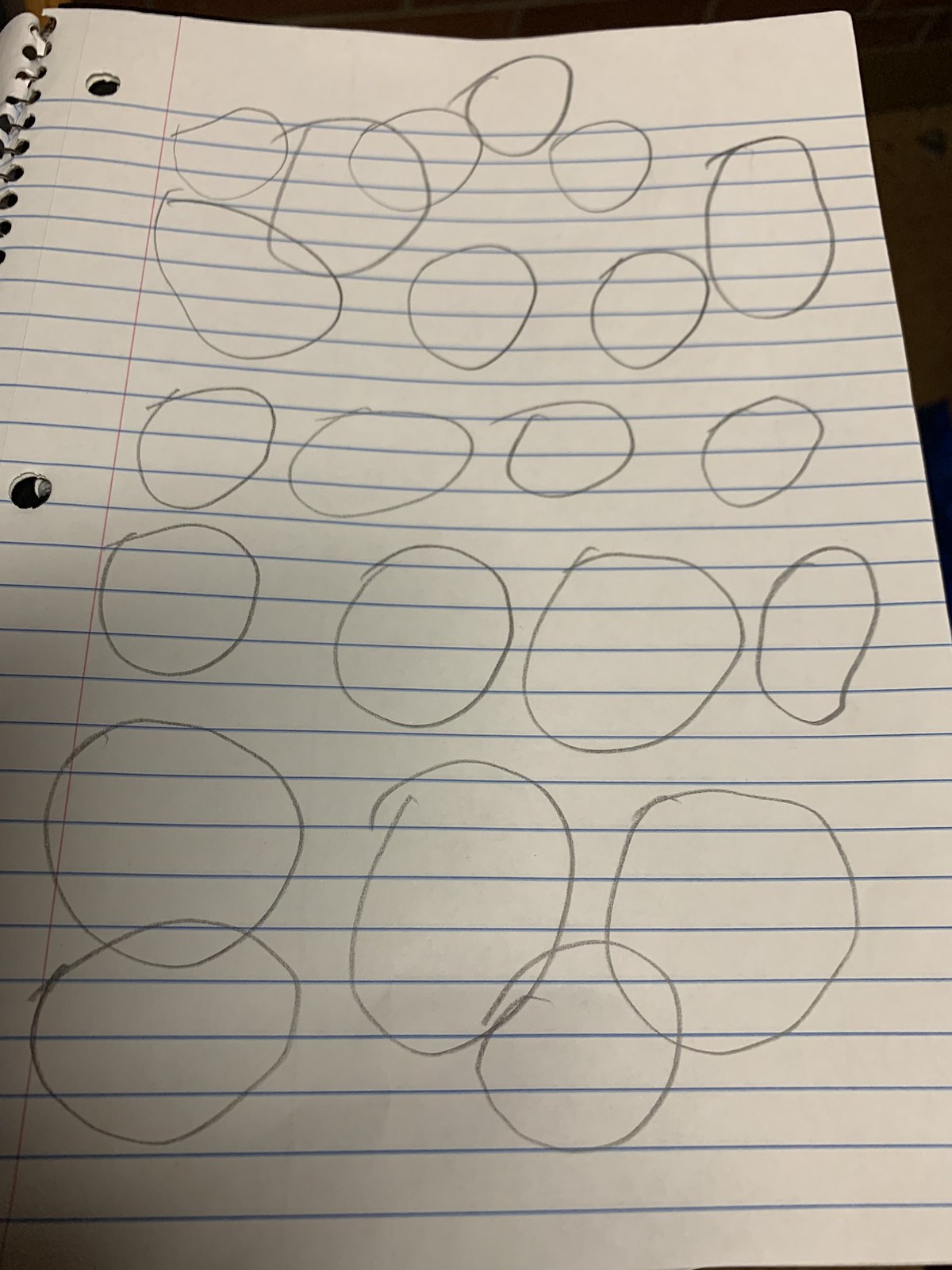A hand-drawn page from a spiral-bound notebook features approximately 22 circles, varying in size from three-quarters of an inch to two inches in diameter. These circles are irregularly shaped, with some appearing oblong or distorted. Several circles overlap or touch, while others stand alone. The artist has carefully avoided drawing in the page's margins. The notebook's spiral binding is visibly damaged, causing the paper to bunch up around the coils and creating the impression that it may not turn or tear cleanly. The page is also hole-punched, suggesting it could be placed into a three-ring binder.